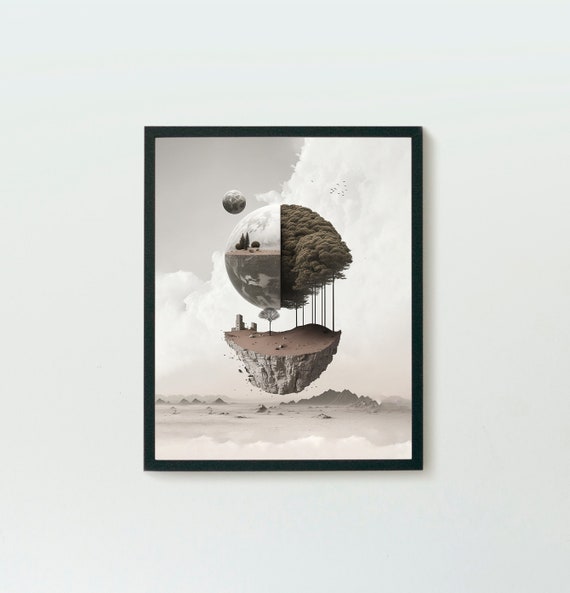This painting, mounted in a simple black frame and hung on a stark white wall, features a surreal and abstract composition, evoking a style reminiscent of MC Escher's work. Central to the image is a large, floating, conical fragment of earth, anchored between treetops on one side and a beach scene on the other. Above this floating landmass hovers a perfectly spherical rock, possibly representing a small moon or distant planet. The backdrop consists of a cloudy sky, with mountains emerging from the mist at the base of the scene. The artwork, primarily rendered in grayscale and muted tones, suggests a fantastical fusion of landscapes, combining elements such as trees, clouds, and an ambiguous globe-like sphere, creating a vision both futuristic and dreamlike.